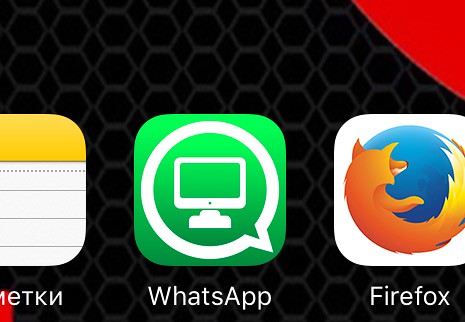This close-up image captures a section of a digital screen, possibly from a computer or a phone. The background is composed of a pattern of grayed hexagons, subtly forming a textured surface that might initially appear solid black. 

In the upper right corner, there is a red triangular shape. Below this, three app icons are arranged horizontally from right to left. 

The first app icon on the right, labeled "Firefox," features a rounded square with a vivid globe and a fox curled around it. The fox is predominantly orange, transitioning into yellow and white at the tail, and has a small black nose. 

The middle icon is the WhatsApp logo, also within a rounded square. It displays a green background and a white speech bubble with the silhouette of a phone handset inside, along with a small protrusion on the lower right edge of the speech bubble. 

The leftmost icon is partially visible, showing the letters "E T K backward N," with a gold section on the top and what appear to be small, dot-like markings. Below these, there are three gray lines against a gray surface.

The overall composition, against the hexagon-patterned background, creates an intricate and visually engaging representation of these digital elements.